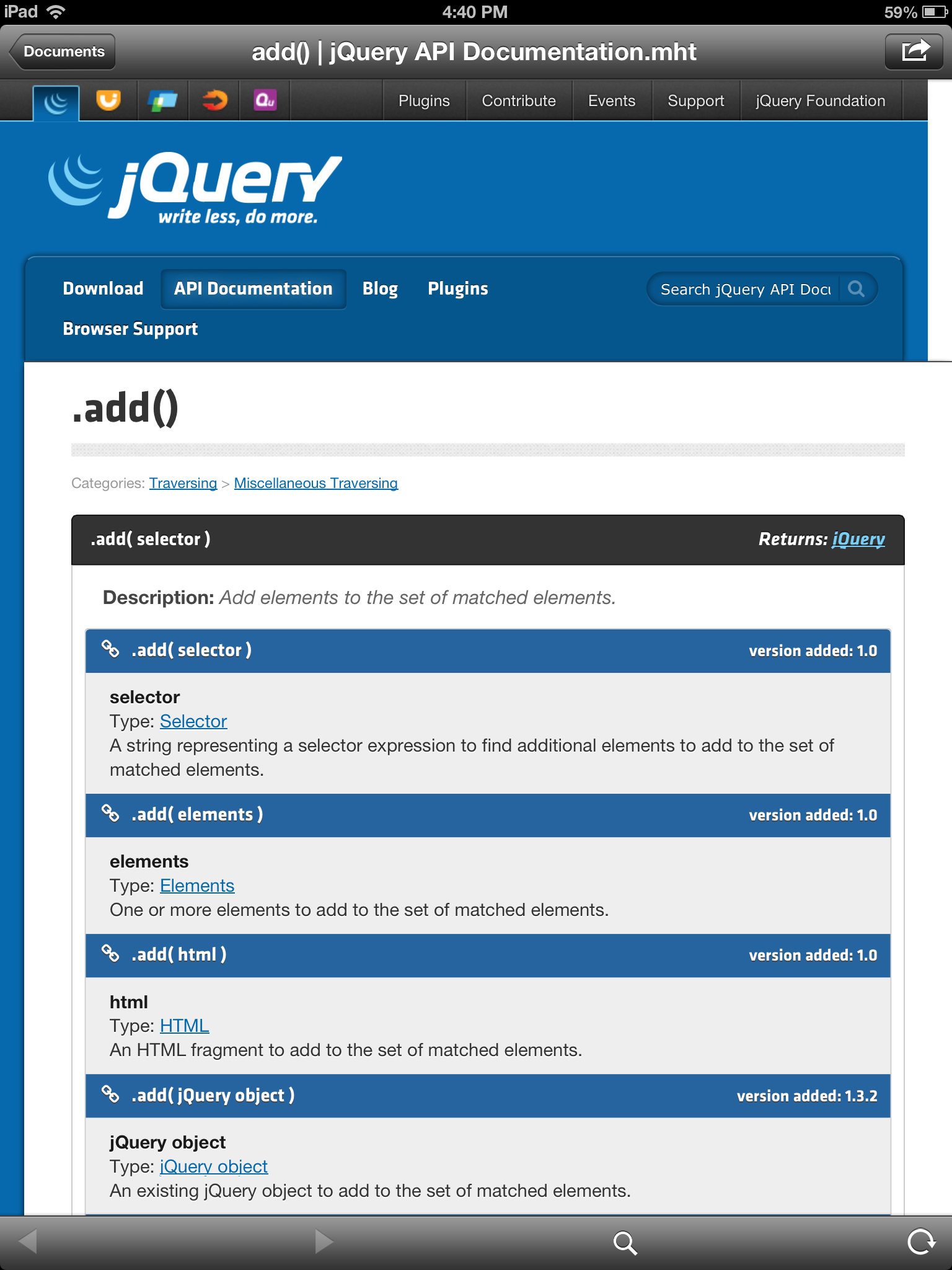Here is a cleaned-up and detailed descriptive caption for the image described:

---

This is a detailed screenshot from an iPad, discernible by the "iPad" label and typical iPad status indicators at the top left corner. The status bar shows the Wi-Fi signal strength, the current time as 4:40 PM, and the battery level at 59%, accompanied by a corresponding battery icon. The top edge of the screen features a black stripe.

The screenshot captures a page of API documentation for jQuery. At the top of the page, there is a navigation link labeled "Documents," along with the title "add() | jQuery API Documentation." Adjacent to this is an icon resembling a right-pointing arrow emerging from a box, possibly indicating a forwarding or sharing option. The page appears to be proprietary content. 

In the documentation section, there are icons representing five different applications. The first is jQuery, followed by a second icon resembling a one-eyed smiley face on an orange shield. Another icon features three rhomboid rectangles arranged in a layered overlay, and a fourth depicts a red and orange gradient circle with a black arrow. The fifth icon shows the letter "Q" with smaller, illegible text beneath it.

A navigational menu with white text on a black background lists options such as "Plugins," "Contribute," "Events," "Support," and "jQuery Foundation." Below this, the page background transitions to blue, displaying the jQuery logo and its tagline, "Write Less, Do More."

The main content area includes a navigation box with a slightly skewed display. Highlighted is the "API Documentation" link in a darker blue bar. Other options include "Blog," "Plugins," "Browser Support," and a search box on the right, partially obscured with the text "Search jQuery API Documentation" and a magnifying glass icon.

Beneath this, the interface returns to a white background with black text, focusing on the ".add()" function within the "Traversing" category. 

Another section in the documentation describes the "add()" function: 
- **Header**: A black background with white text reads ".add() function - Category: Traversing, Miscellaneous."
- **Details**: 
  - **Description**: "Add elements to the set of matched elements."
  - **Selectors**: 
    - **.add( selector )** - Blue text header with white text on dark blue background. Introduced in version 1.0, it includes black text on a gray background stating: "A string representing a selector expression to find additional elements to add to the set of matched elements."
    - **.add( elements )** - Same header style, details: "One or more elements to add to the set of matched elements." Introduced in version 1.0.
    - **.add( HTML )** - Details: "An HTML fragment to add to the set of matched elements." Introduced in version 1.0.
    - **.add( jQuery object )** - Details: "An existing jQuery object to add to the set of matched elements." Introduced in version 1.3.2.

Each section consistently follows the white text on a dark blue header, with corresponding black text on a gray background for descriptions and parameters.